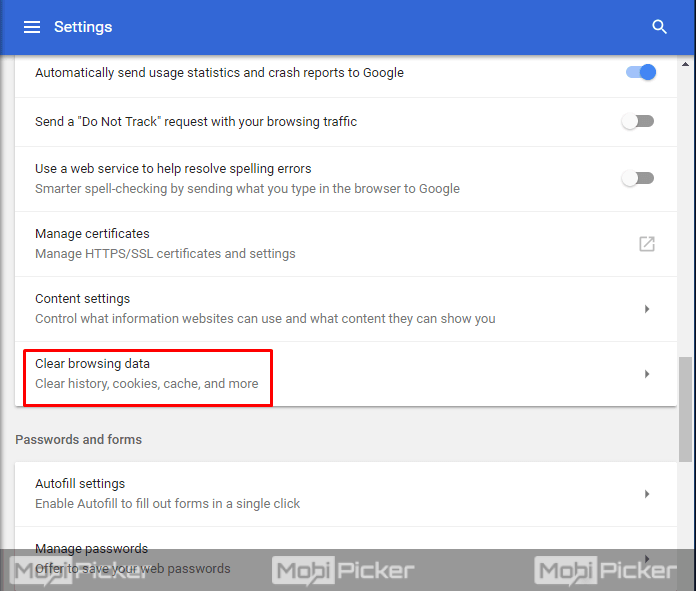The image depicts a settings page interface, dominated by a blue header that stretches horizontally across the top of the image. Within the blue bar, the word "Settings" is prominently displayed in white font with an initial capital "S," and is accompanied by an icon showing three horizontal lines, situated next to the text.

Below the header, the first section titled "Automatically send usage statistics and crash reports to Google" is visibly activated, indicated by a toggle switch that is turned on. Following this, the second option, "Send a 'Do Not Track' request with your browsing traffic," is presented, with its toggle switch in the off position. The third setting, "Use a web service to help resolve spelling errors," is similarly toggled off.

The subsequent section labeled "Manage certificates" includes a subtext in gray font that reads "Manage HTTPS/SSL certificates and settings." Farther down, there is a section titled "Content settings," followed by an additional setting critically highlighted with a red triangle next to "Clear browsing data." This section offers further clarification, stating, "Clear history, cookies, cache, and more."

All elements combine to provide a comprehensive overview of various browser settings and functionalities.